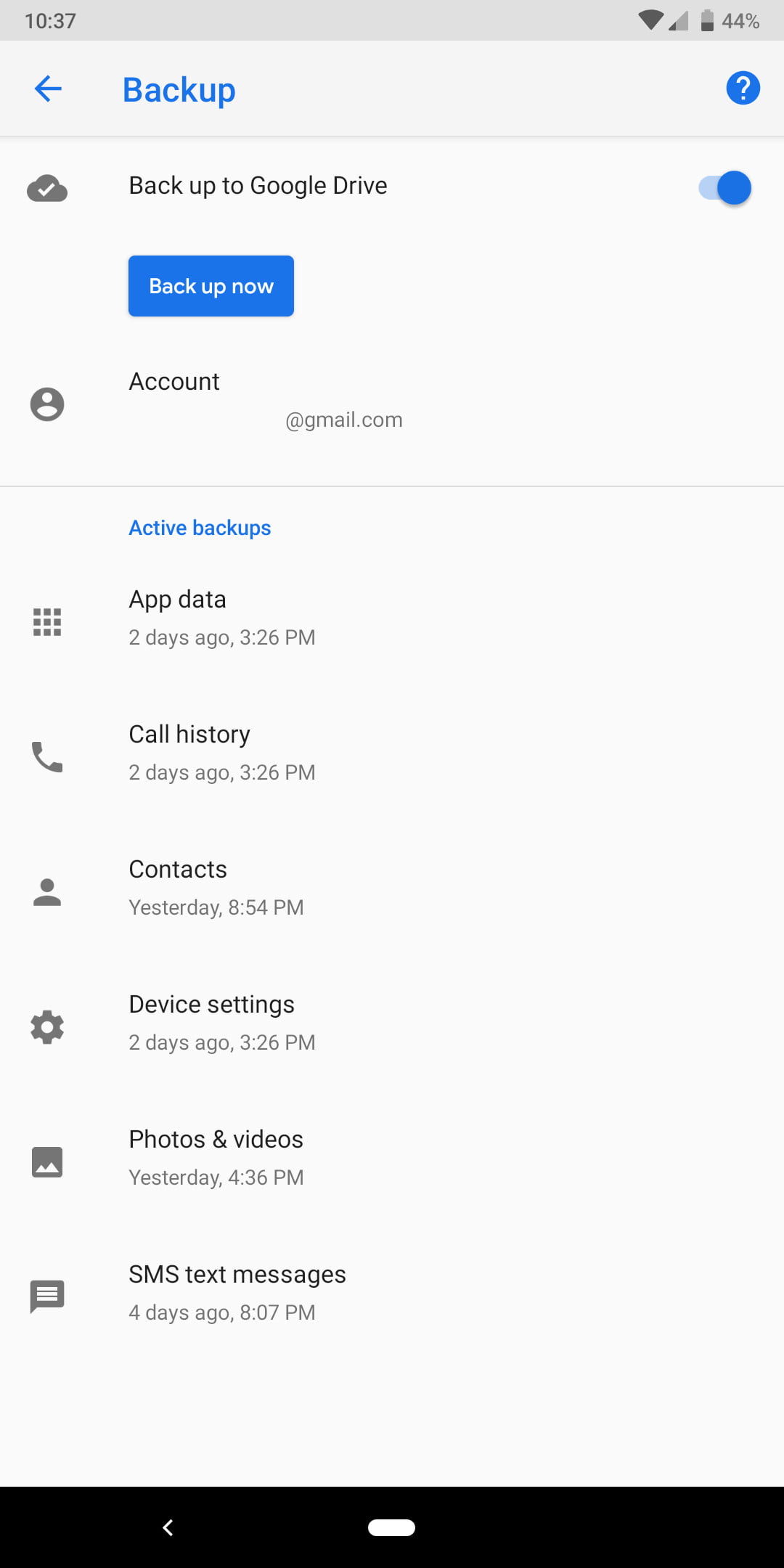This image is a screenshot taken from a cell phone, displaying a backup settings screen. At the very top, a thin gray border frames the status bar, where the time is displayed on the top-left in black as "10:37." On the right side of the status bar, icons indicate the phone's connectivity and battery status, including an upside-down Wi-Fi triangle with one bar, and the battery level at 44%.

Below the status bar, blue text on the left reads "Backup," accompanied by a blue arrow pointing left. To the right of this text is a blue circle with a white question mark inside it. Moving further down, there is a rectangular section containing the following text: "Back up to Google Drive." Adjacent to this text, within a blue rectangle, are white letters that spell "Back up now." To the right of this rectangle, there's a blue toggle switch that is currently turned on.

Below this segment, the text "Account" appears with the placeholder "[your email address]@gmail.com." A light gray border separates this section from the one below it. Underneath, the text "Active backups" is displayed in blue. Listed in sequence from top to bottom, the categories for backup include: App Data, Call History, Contacts, Device Settings, Photos and Videos, and SMS Text Messages. Finally, the bottom of the screenshot is framed by a black border.